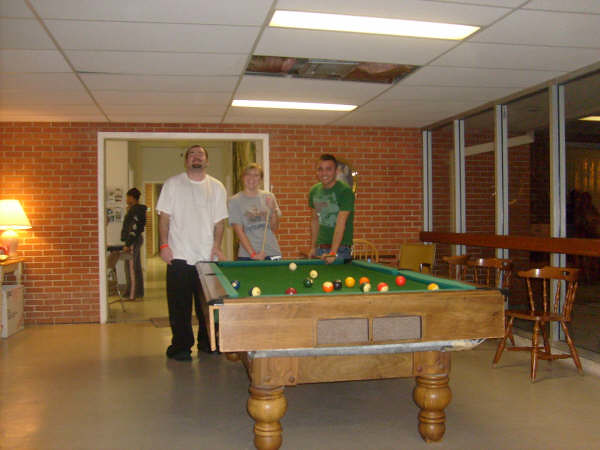In this indoor scene, a group of three young people, likely in their late teens or early 20s, are gathered around an old-fashioned brown wooden pool table covered in green felt. The pool table has large, rounded legs and is filled with multicolored pool balls. The room has a somewhat cozy but slightly dim ambiance, with overhead white drop ceiling tiles and a section with two lights and a missing tile between them. 

In the background on the right side, four large glass windows stretch from floor to ceiling, with three small brown chairs in front of them and a dark horizontal wooden beam two-thirds of the way down. The windows meet a brick wall on the left side, which has a desk with a lamp turned on about two inches in from the wall's edge, and a yellow chair situated in the corner. A large opening with a white border is visible on the left, leading to another room, where a person's silhouette can be seen.

In the center of the image, three friends stand on the far side of the pool table, looking towards the camera. On the left, a man with a goatee, short brown hair, and glasses stands wearing a long white t-shirt, black pants, black shoes, and a red wristband. Next to him, a woman with blonde hair in a fitted gray t-shirt with a graphic on it holds a pool cue diagonally across her body. To her right, another man with short dark hair, tanned skin, and a green graphic t-shirt leans on the pool table with his left hand, his blue jeans partially visible.